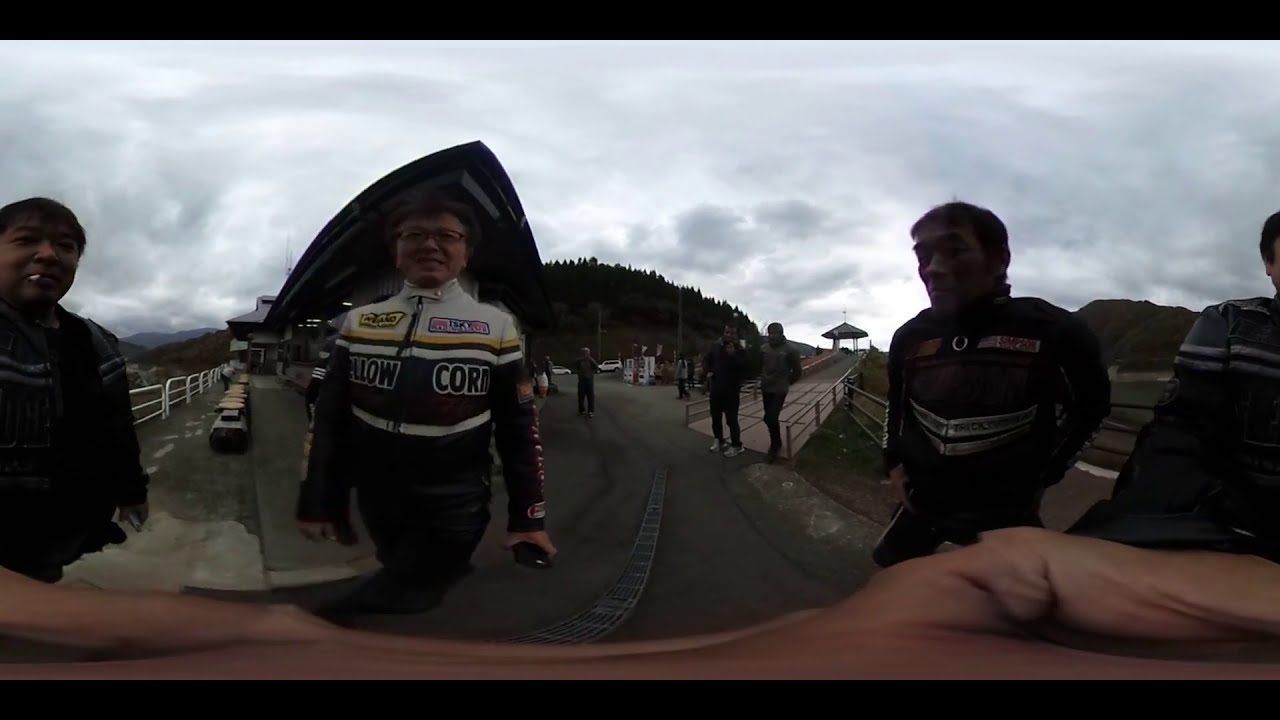This outdoor photograph depicts a somewhat distorted, panoramic view of a group of people on an overcast day with dark grey skies. The image, altered by a special effect, has a stretched appearance, contributing to its unique and surreal feel. Three men are seen prominently in the foreground, accompanied by part of a fourth man on the side. All appear to be of Asian descent and are dressed in sports outfits, possibly for a competition. 

The first man, situated leftmost, sports a black jacket with grey stripes, a black shirt, and has his hands in his pockets, with a white cigarette in his mouth. The second man, standing next to him, wears a distinctive racetrack suit with black pants, a white belt, and a black and white jacket featuring a yellow and black stripe in the middle, adorned with multiple logos and texts. The third person, wearing glasses, is clad in a zip-up black and white top with various writings and logos, including the phrase "Yellow Corn" in black letters. The fourth man is only partially visible on the edge of the image.

The background features more people standing and walking, cars parked in the distance, a covered walkway that rises to the right, and a building off to the left. Tall, forested mountains stretch across the horizon, with numerous trees adding to the serene ambiance of the overcast setting. The photograph also includes hands apparently holding the camera, visible at the bottom corners, adding to the panoramic and immersive effect of the image.